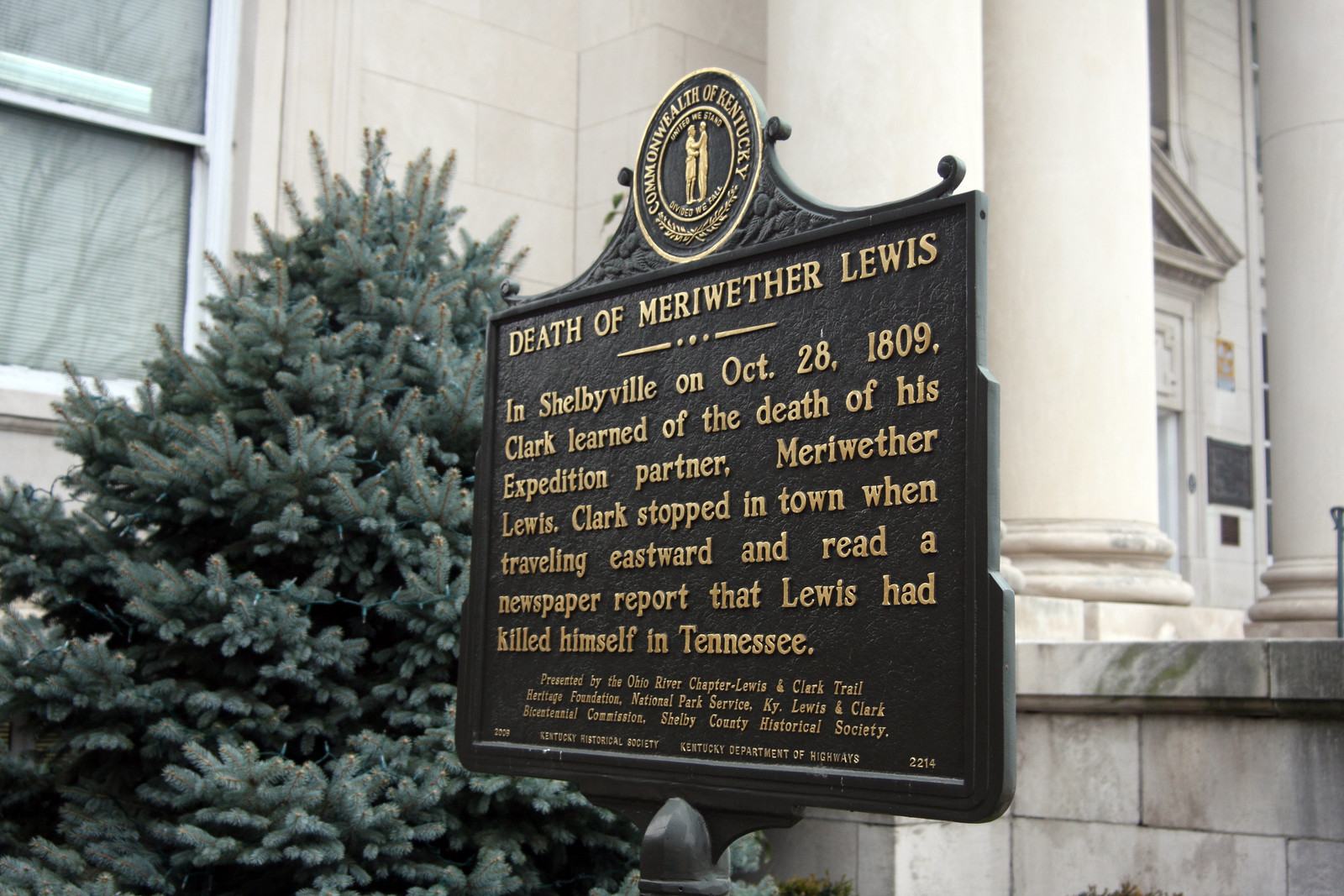The image captures a historical plaque prominently displayed outside a white stone building characterized by its large white columns. In the vicinity of the plaque, there is a distinctive coniferous tree, likely a blue spruce, adorned with some unlit Christmas lights, and a nearby window. The building itself exudes a sense of grandeur, suggestive of an ornate state house. The plaque, cast in bronze with raised gold letters, stands out as the main focus of the image. At the top of the plaque is a circular seal that reads "Commonwealth of Kentucky," featuring an emblem with two figures. The primary text on the plaque reads: "Death of Meriwether Lewis. In Shelbyville on October 28, 1809, Clark learned of the death of his expedition partner, Meriwether Lewis. Clark stopped in town when traveling eastward and read a newspaper report that Lewis had killed himself in Tennessee." Additional smaller text indicates that the plaque was presented by someone, in conjunction with the Shelby County Historical Society. No people are present in the scene, highlighting the solemn historical significance of the site.